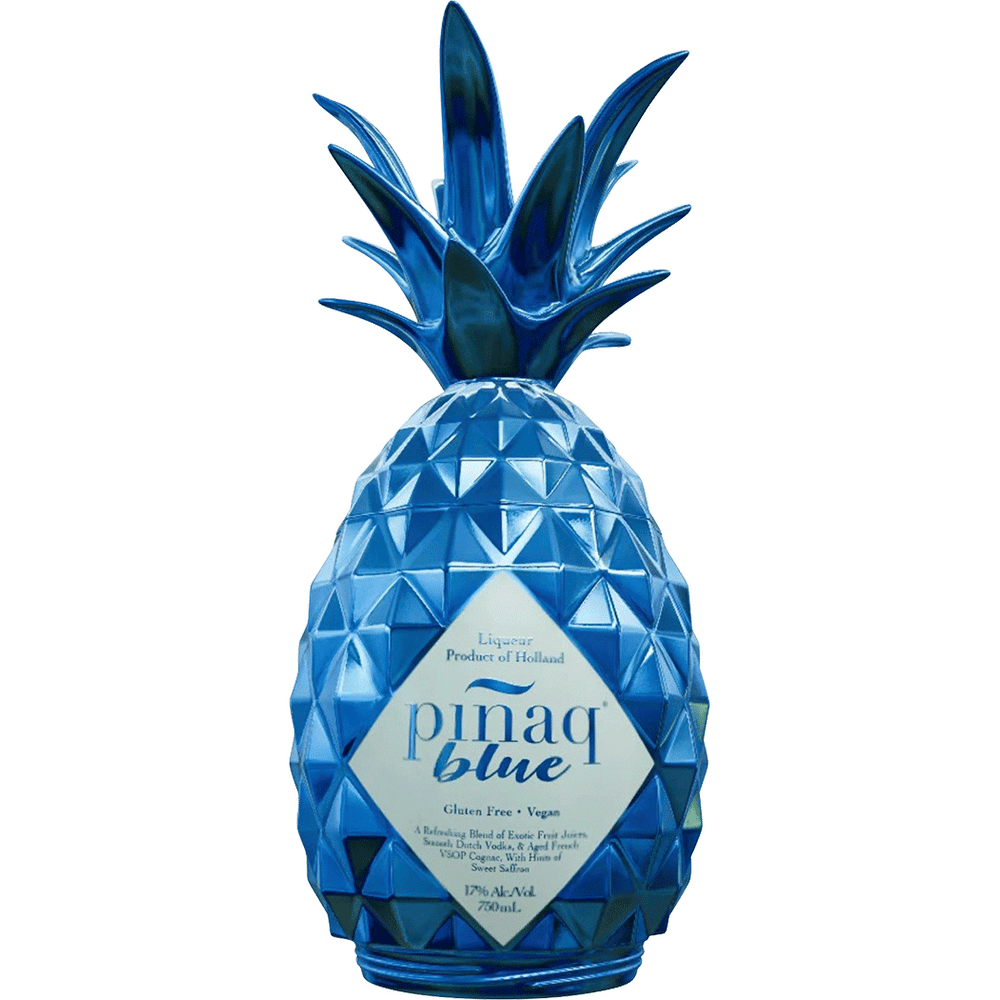The image depicts a creative liquor bottle shaped like a pineapple, with a detailed design in varying shades of metallic blue. The bottle features a darker blue hue on the top, which forms the lid resembling pineapple leaves, and a lighter blue body with intricate point and indentation patterns simulating a pineapple's texture. The bottle is adorned with a white, diamond-shaped label, which includes blue text. The label reads "Liqueur Product of Holland, Pignac Blue," and highlights that the product is "gluten-free" and "vegan." Further text indicates it is a "refreshing blend of seasonal Dutch vodka and fruit juices," although parts of the description are not entirely legible. The bottom of the label specifies that the alcohol content is "17%," and the bottle holds "750 milliliters." The background of the image is plain white, making the striking design of the blue pineapple bottle the focal point. This unique and intriguing bottle design suggests it could be marketed online.